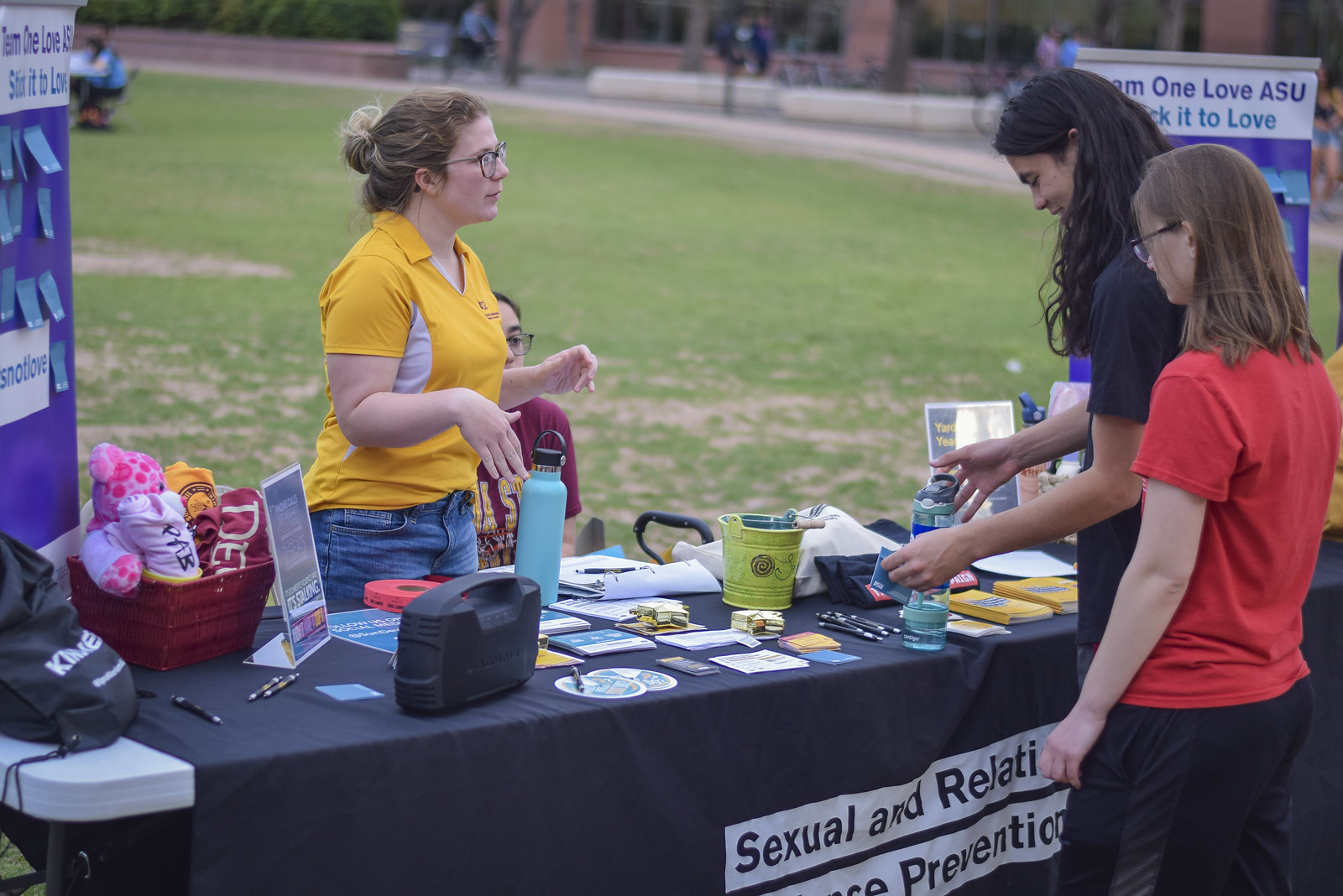The image captures a group of individuals gathered around a long table covered with a blue tablecloth. The setting appears to be a large grassy field in front of a brick building, with a road or pathway visible in the background. The table is part of a daytime outdoor event focused on sexual and relationship prevention awareness. The tablecloth features text that reads "sexual and relationship prevention," although part of the writing is cut off.

On the table, there are various items such as pamphlets, stickers, pens, raffle tickets, and brochures, indicating that information and possibly merchandise like t-shirts are being distributed. A blue thermos and a red basket filled with plush dolls or shirts add to the display. Several laminated cards or flyers are also visible.

Behind the table, a lady in a yellow polo shirt with white accents, glasses, and a bun is present. Another woman in a red shirt and glasses stands next to her, wearing black track pants. On the opposite side of the table, two young girls—one in a red shirt and another in a dark shirt—are seen engaging with the materials laid out. There’s also a young man with long brown hair observing the setup. Overall, it depicts a community outreach effort aimed at raising awareness on important social issues.